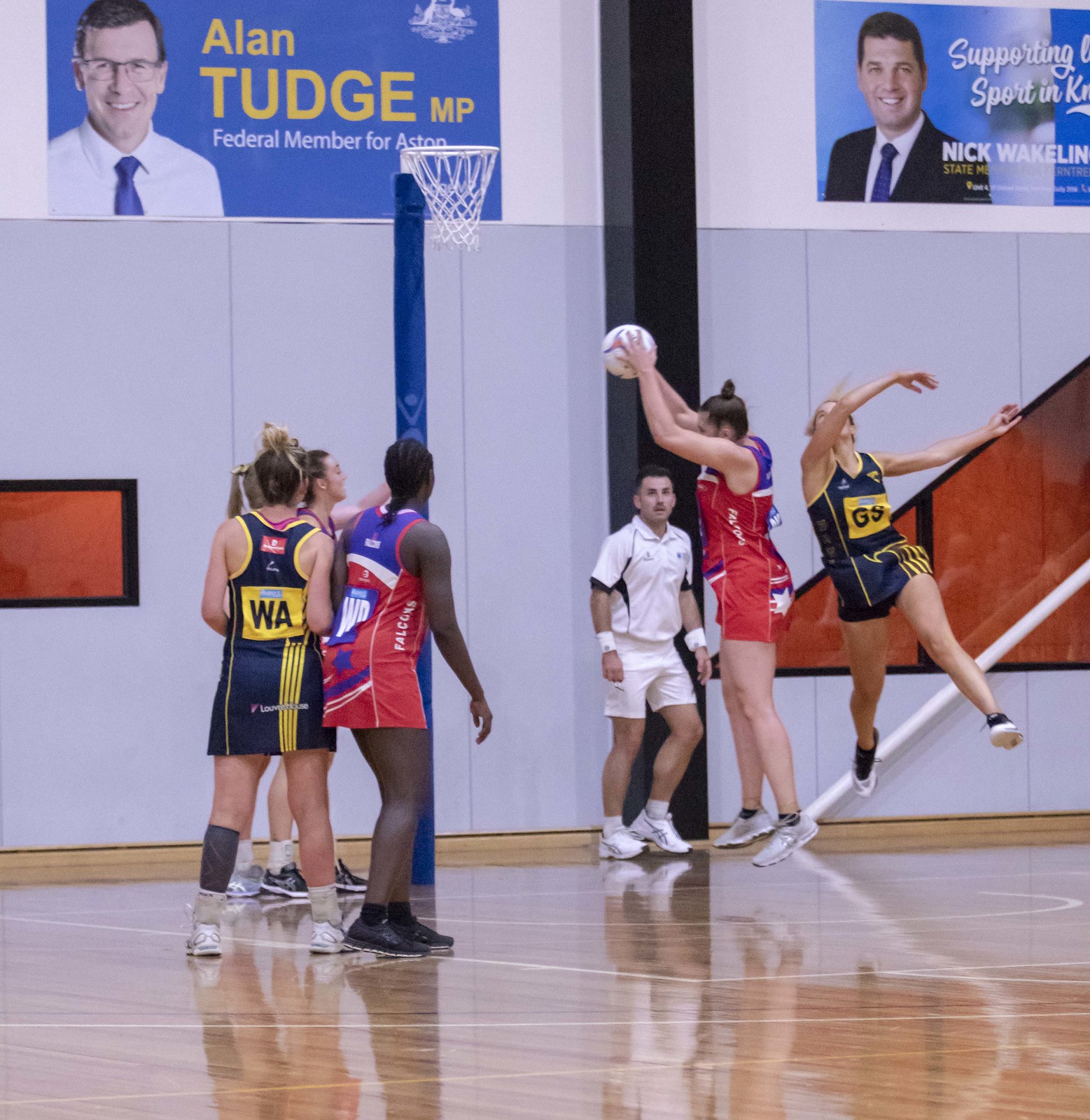The image depicts a dynamic scene of a netball game played by young female athletes on a polished wooden court. At the center of the action, a black woman in a short sports skirt with red, blue, and white collars, and sleeveless black trainers, stands with her back to the camera. She is observing her teammate, who is clad in a red, white, and blue uniform with grey trainers, as she leaps into the air, arms raised to catch a white ball patterned with triangles.

To the right of the jumping player, another competitor dressed in grey and yellow uniform arches her arms to the right, legs spread apart. On the left side of the image, two girls—also in grey and yellow attire—stand on the ground, looking towards the ongoing play. 

In the background, a coach or referee, wearing a white polo shirt, white wristbands, white shorts, and white trainers, keenly watches the game. The court features a glossy wooden floor marked with white stripes, a blue cylindrical pole with a hoop and white net positioned in the center.

The court is framed by grey walls adorned with posters. One poster on the left displays Alan Tudge MP, the federal member for Aston, set against a yellow background. To the right, another sign promotes Nick Wakelin, with the text "supporting sport in" partially visible. The gymnasium's windows, bordered in black and glowing orange from the inside, add to the setting of this vibrant sports event. Both teams exhibit distinct uniforms, with one team in blue and yellow outfits featuring identifiers like "WA" and "G9," while the other team wears blue, white, and red, adorned with stars and letters such as "MP" or "WP."